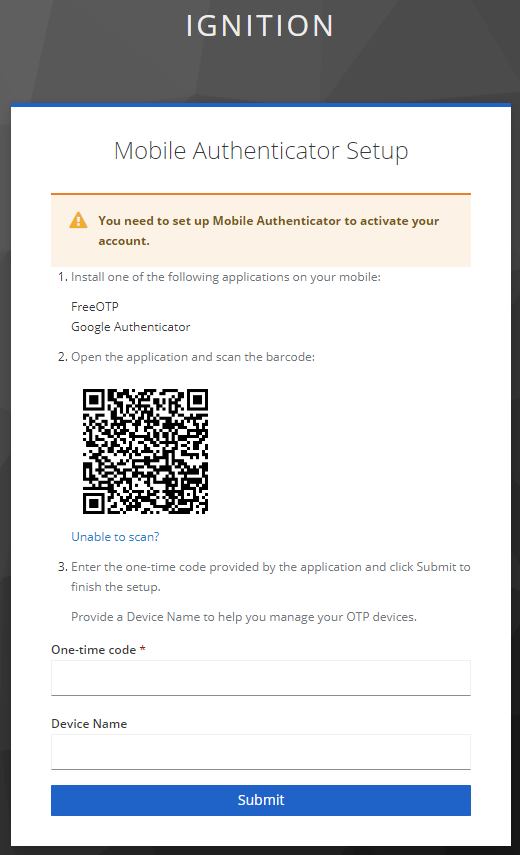Dialogue box for mobile authentication app:

---

**Header:**
- The top section features a subtle grayish design background.
- Centered at the very top is "IGNITION" in white all-caps lettering.

**Main Content:**
1. **Primary Dialogue Box:**
   - A white background with a thin blue line at the top.
   - Text: "Mobile Authenticator App" in gray.

2. **Alert Box:**
   - A highlighted pale red dialogue box with a red line at the top.
   - On the left, an orange triangle with a white exclamation mark.
   - Text inside reads: "You need to set up a mobile authenticator to activate your account" in a brownish-gray color.

3. **Instructions:**
   - Text: "1. Install one of the following applications on your mobile:" followed by a colon.
   - Options:
     - "FreeOTP" (OTP in capitalized letters)
     - "Google Authenticator"
   - Text for "Installing" in gray below the first instruction.
   
   - "2. Open the authentication application and scan the barcode:" in gray.
   - A black and white QR code with three positioning squares at the top-right, top-left, and bottom-left corners.
   - Under QR code: "Unable to scan?" in blue, acting as a link.

   - "3. Enter the one-time code provided by the application and click SUBMIT to finish the setup:" in gray.
   - "Provide a device name to help you manage your OTP devices."

4. **User Input Fields:**
   - Label: "One-Time Code*" in black with a red asterisk indicating it’s required.
   - An empty text box for the one-time code.
   - Label: "Device Name" in dark gray with an empty text box underneath.

**Footer:**
- At the very bottom, a blue "SUBMIT" button is placed directly under the text boxes.